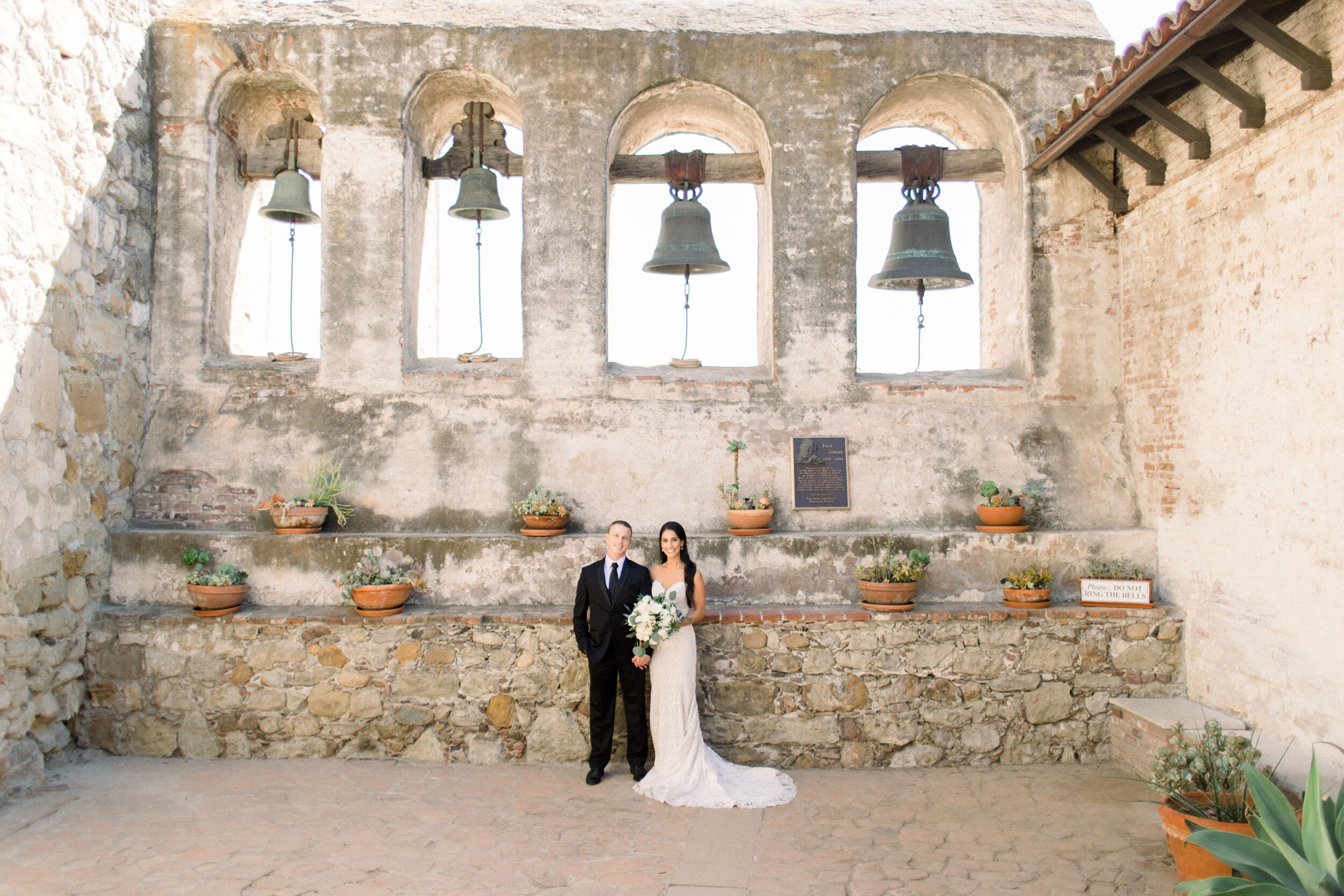In this brightly lit outdoor photograph, a bride and groom stand in the courtyard of a grand, old building with Mediterranean-style architecture. The backdrop shows four large, traditional church bells hanging in arched openings, each with a rope for ringing. The couple is framed by lush greenery in various potted plants and terracotta wide bowl-shaped planters, arrayed across two stone terraces behind them. The groom, positioned on the left, is dressed in a solid black suit with a black tie and a white collared shirt, and has short dark blonde hair. He beams beside the bride, who wears a stunning strapless white gown with a trailing train and clutches a bouquet of white flowers adorned with greenery. She has long dark hair cascading over her shoulder. The courtyard is bathed in sunlight, with a shaft of light falling diagonally across the stone wall on the left. The reddish cobblestone floor adds to the rustic charm, with additional plants framing the sides and a bench along the wall, lending a picturesque and serene ambiance to this celebratory moment.